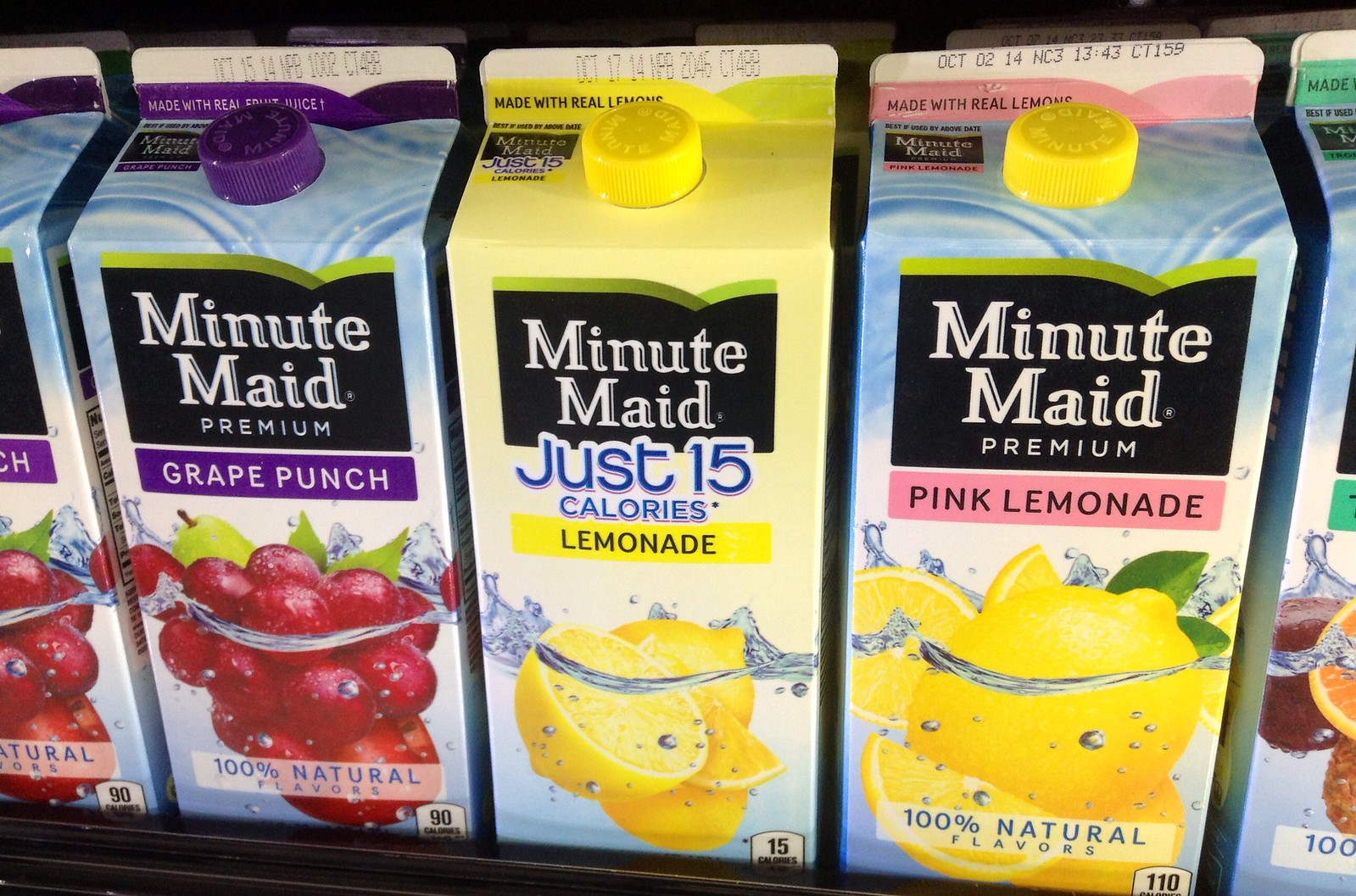This is a close-up photograph of Minute Maid cartons in the refrigerated section of a grocery store. The image prominently features three fully visible cartons and part of two others. On the left, a Minute Maid Premium Grape Punch carton has a purple cap and showcases a close-up of red and green grapes at the bottom, alongside the text "100% Natural Flavors". The carton’s upper portion is blue. In the middle, the Minute Maid Just 15 Calories Lemonade carton has a yellow cap and a submerged lemon design, with a yellow upper portion. To the right, the Minute Maid Premium Pink Lemonade carton, also with a yellow cap, features partly submerged lemons and a dark green leaf, with "100% Natural Flavors" written on it, and it has a blue upper portion. The cartons are rectangular, made of cardboard, taper into a point at the top with cylindrical caps, and display expiration dates and lot numbers on the upper flaps. The scene captures them neatly arranged and awaiting purchase.